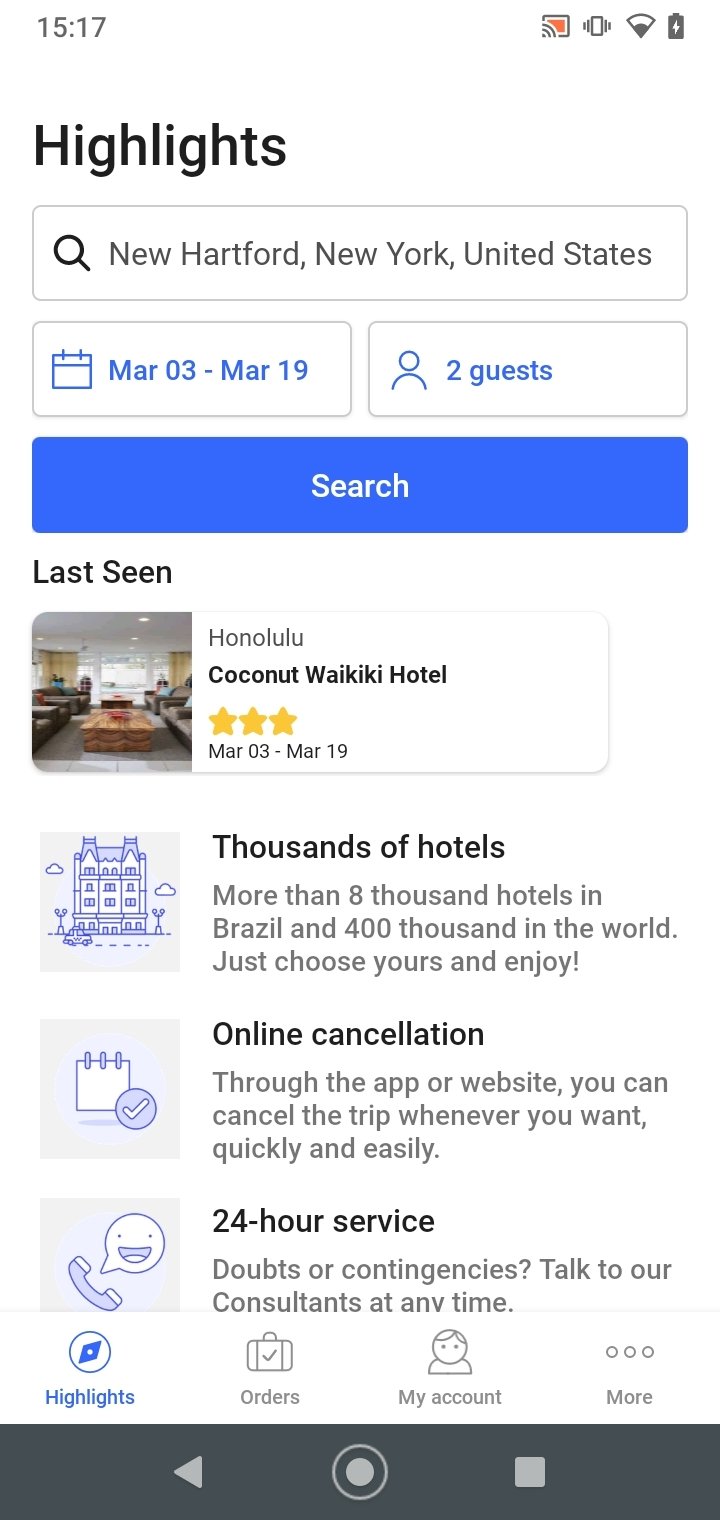Here's a cleaned-up and detailed caption for the screenshot:

---

The screenshot displays a web interface captured at 15:17, featuring standard indicators for battery and network status on the upper right. 

At the center, there is a search query in bold black capital letters "H," with a location specified as New Hartford, New York, United States. The search settings indicate travel dates from March 3rd to March 19th. 

The interface prompts users to click the blue search button to proceed. Below, a series of information snippets are visible:
1. **Last Seen:** The Waikiki Hotel in Honolulu's Coconut Walk area, rated three stars.
2. **Hotels Options:** Over 8,000 hotels in Brazil and 400,000 globally, providing a vast selection for users to choose from and enjoy.

The image includes various icons and pictures:
- An etching of a castle representing numerous hotel options.
- A picture of a hotel room corresponding to the Waikiki Hotel.
- An icon depicting a webpage for the online cancellation feature.
- A phone icon denoting 24-hour service accessibility.

The metadata highlights the convenience of flexible online cancellation through the app or website, and 24-hour support for any doubts or contingencies, encouraging users to contact consultants at any time for assistance.

---